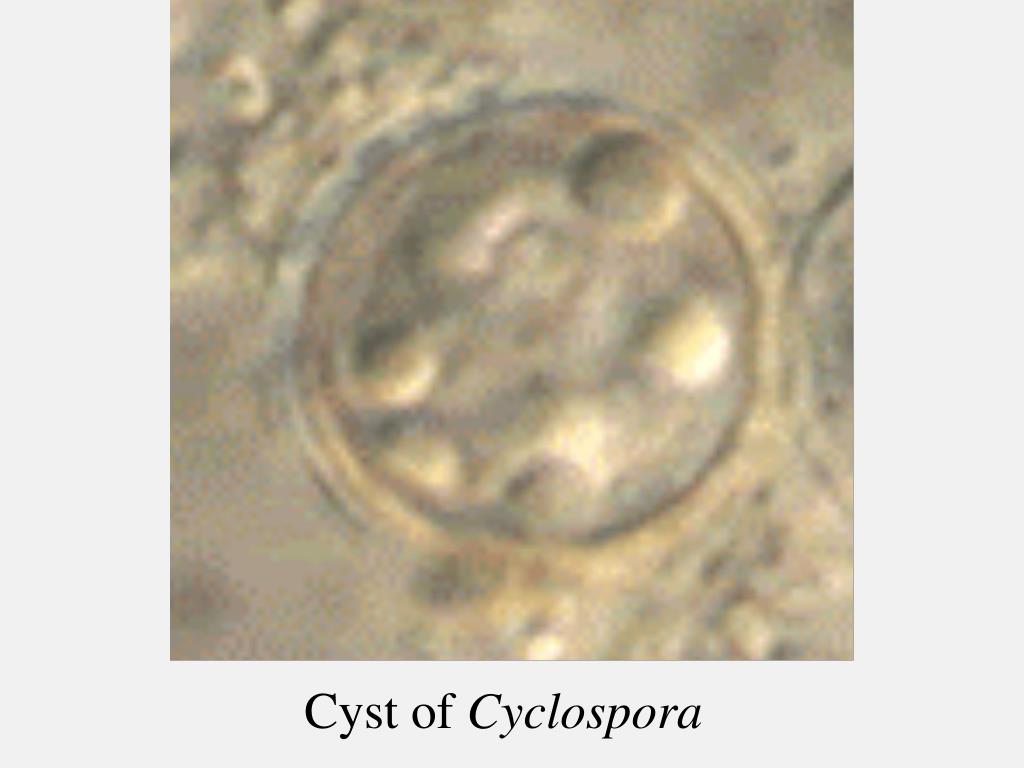This image portrays a microscopic close-up of a cyst of Cyclospora, set against a solid light gray background. The focal point is a central square framed in brown and beige hues, with darker brown shading in the upper right and lower left corners, and lighter textured lumps of beige and brown in the upper left and lower right corners. Encased within this square is a prominent circular ring with several larger, dotted lumps inside, varying in shades from dark brown to beige. Notably, to the right of the central circle, another partial circle intersects into view. This entire portrayal mirrors the intricate, scientific aesthetics of cellular structures, and beneath the image, the text "cyst of Cyclospora" is displayed in bold, black lettering.